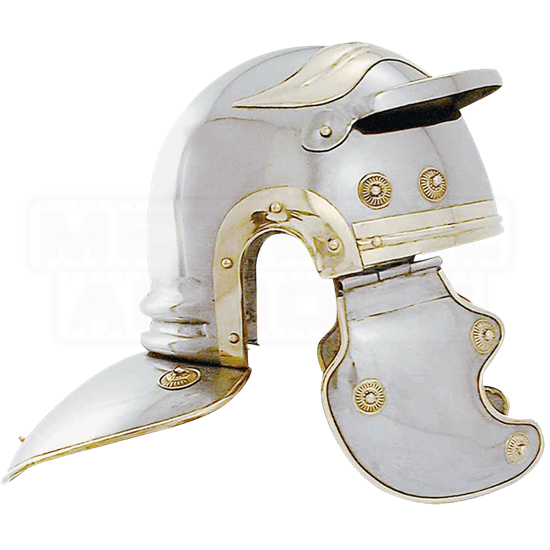This image features a polished, metal helmet characteristic of a knight in shining armor from medieval times. The helmet gleams in a shiny chrome finish and is embellished with intricate designs and accents. Across the top, a lighter silver wave design gracefully dances, while a gold accent adds a touch of elegance. The front of the helmet features two brownish circles akin to rivets, adding a touch of ruggedness.

On either side, the ear protection flaps stand out, exhibiting three round golden rivets each that resemble small shields. These flaps protect the sides of the face, with the ear area accentuated by a shiny chrome trim that loops around, leaving the ears exposed.

The back of the helmet extends outwards with an additional flap, designed to rest on the shoulders and protect the neck area. This back flap also showcases a brown metal circle for added detail. Overall, the helmet is a strikingly detailed piece, capturing the essence of medieval warfare and knightly grandeur against a pure white background.